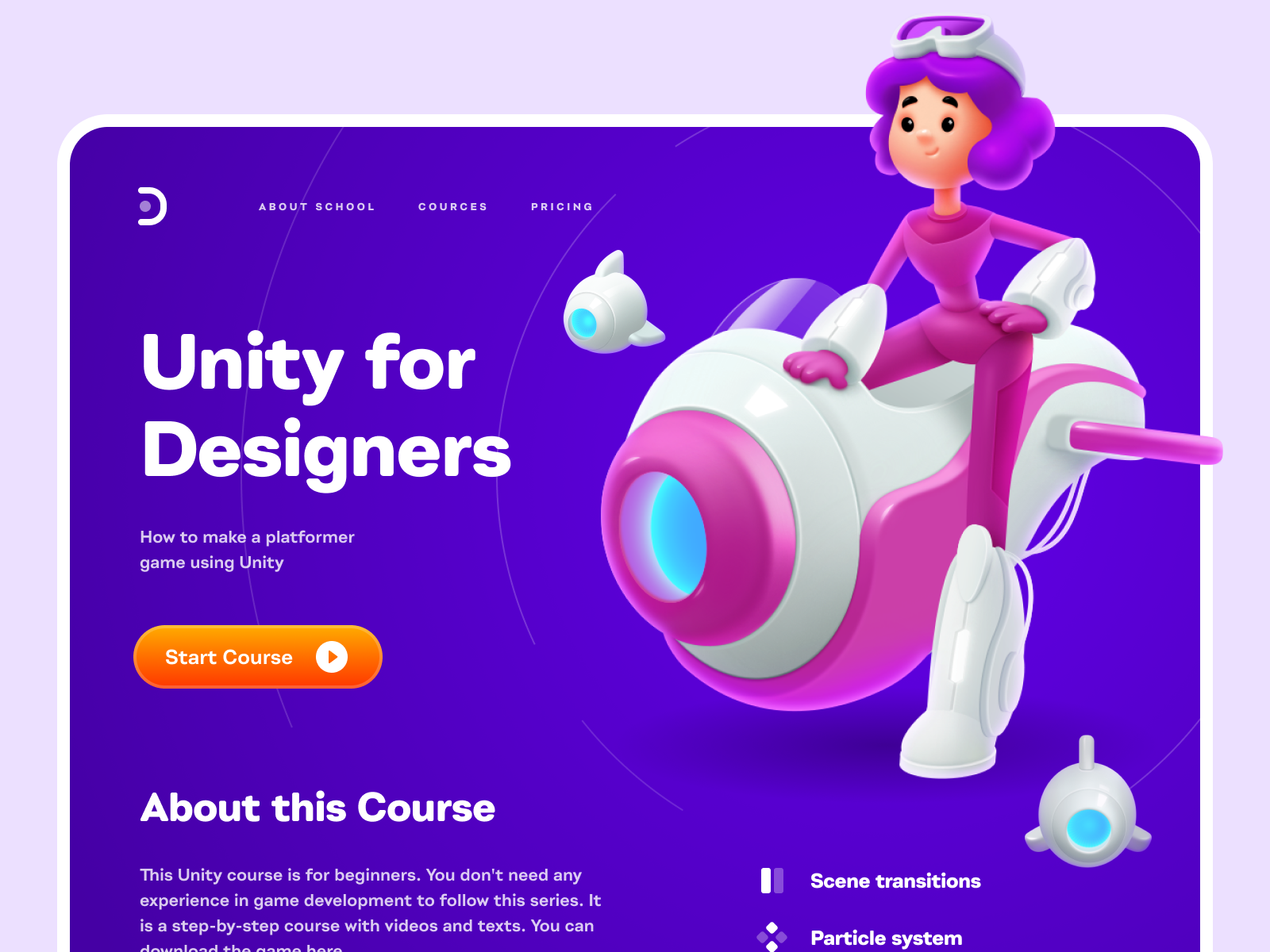The image features a light background with a gradient of purple on the outer edges transitioning to white in the central area, and then back to purple in the innermost section. On the top left, there is a prominent white "D" symbol. Across the top of the image, various terms such as "apart school," "causes," and "pricing" are displayed.

Central to the image is the text "Unity for Designers: How to Make a Platformer Game Using Unity," indicating that this is a Unity webpage designed for aspiring game designers. Below this main title, on the left side, is an orange-shaded rectangular button with the label "Start Course," featuring a play icon to commence the course. 

At the bottom, there is a detailed description stating, "About this course: This Unity course is for beginners; no prior experience in game development is required. It is a comprehensive step-by-step guide with both videos and text. You can download the game here." 

On the bottom right side, there are options like "scene transition" and "particle system." To the right of the main text is an illustrative drawing presumably created with Unity. The drawing depicts a female character with purple hair and glasses, dressed in a pink and white protective outfit with white boots. She is driving a futuristic white and pink space vehicle.